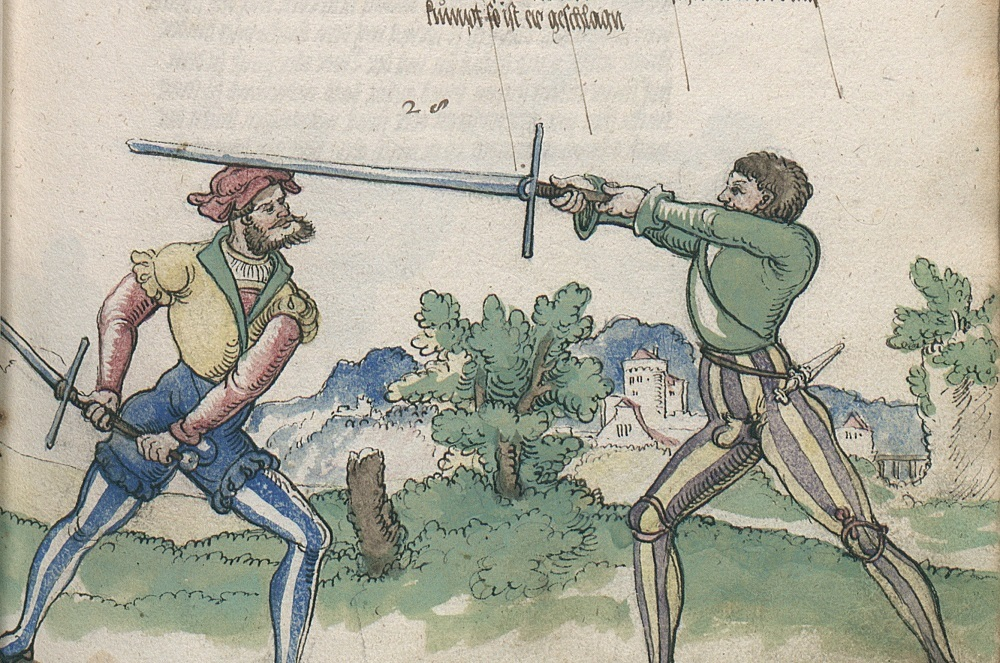In this detailed cartoon-style illustration, set against a backdrop that features a castle-like building, trees, and distant mountains, two Caucasian men are depicted engaging in a medieval duel with swords. The man on the viewers' right is wearing a green long-sleeve shirt paired with striking purple and yellow striped tights. He faces the male figure on the viewers' left, holding a long silver sword that gently touches the top of the other's head, as if knighting him. The man on the viewers' left, who faces to the right, sports a distinctive red bonnet atop his head. His attire includes a yellow short-sleeve shirt with puffy sleeves, a green collar, and a middle section, layered under a red long-sleeve shirt. He also wears blue shorts with puffy bottoms, and white and blue leggings. The scene is complemented by cursive brown text at the top of the image, which appears to be part of an old children's book or illustrated manuscript. The detailed and colorful clothing, combined with the historical setting and the engaged duel, conveys a rich and dynamic representation of a medieval tableau.